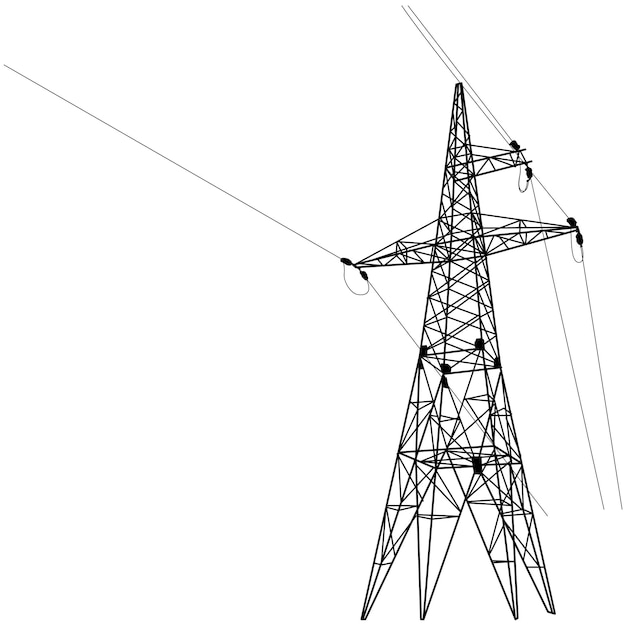This black-and-white drawing depicts a simplistic yet detailed sketch of a tall electric tower. The tower is a long, triangular conical structure composed of numerous rods arranged in triangular and diagonal patterns. Additional features include small square boxes at various levels and a trapezoidal structure near the peak. The electric tower is drawn with the power lines emanating from near the top, winding and extending downward towards the bottom part of the image, where they remain unattached to anything. The entire composition is set against a completely white background, highlighting the stark black lines of the tower and the power lines. This image resembles a sketch rather than a photograph, emphasizing the bare essentials of the electric tower and its associated components.